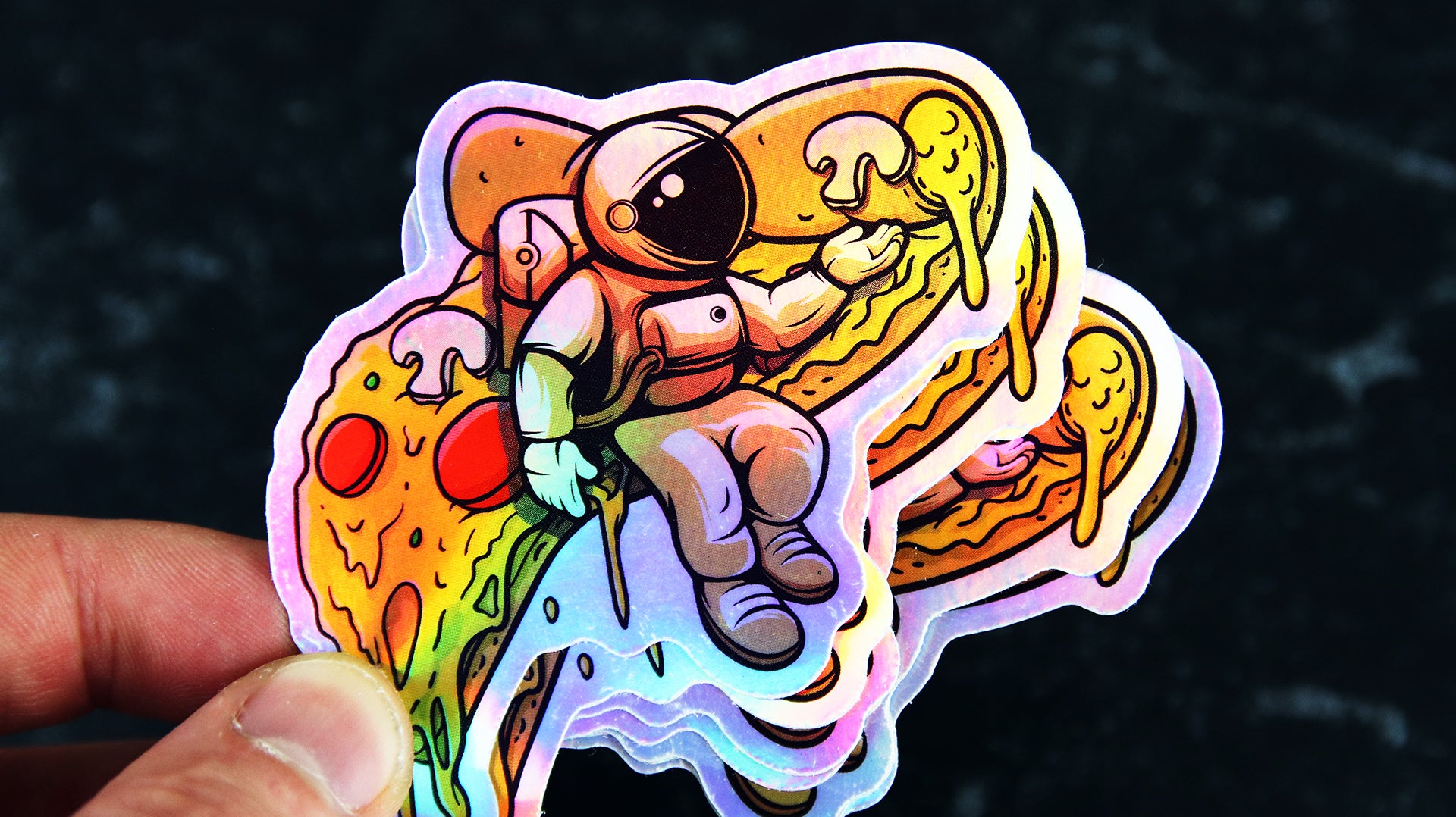This photograph captures a partial view of a person's thumb and index finger, situated in the bottom left corner, holding a stack of at least five stickers, all identical. The stickers depict a detailed, hand-drawn or computer-generated image of an astronaut in a full spacesuit with a white helmet featuring orange and yellow stripes and a black faceplate. The astronaut is seated atop a slice of pizza with cheese melting off the edges. The stuffed crust visibly oozes cheese, and the pizza is topped with pepperoni, mushrooms, and small green bits. The astronaut appears to be either tossing or catching one of the mushrooms. The background of the stickers is black, highlighting the vibrant colors of the pizza and the astronaut's suit.